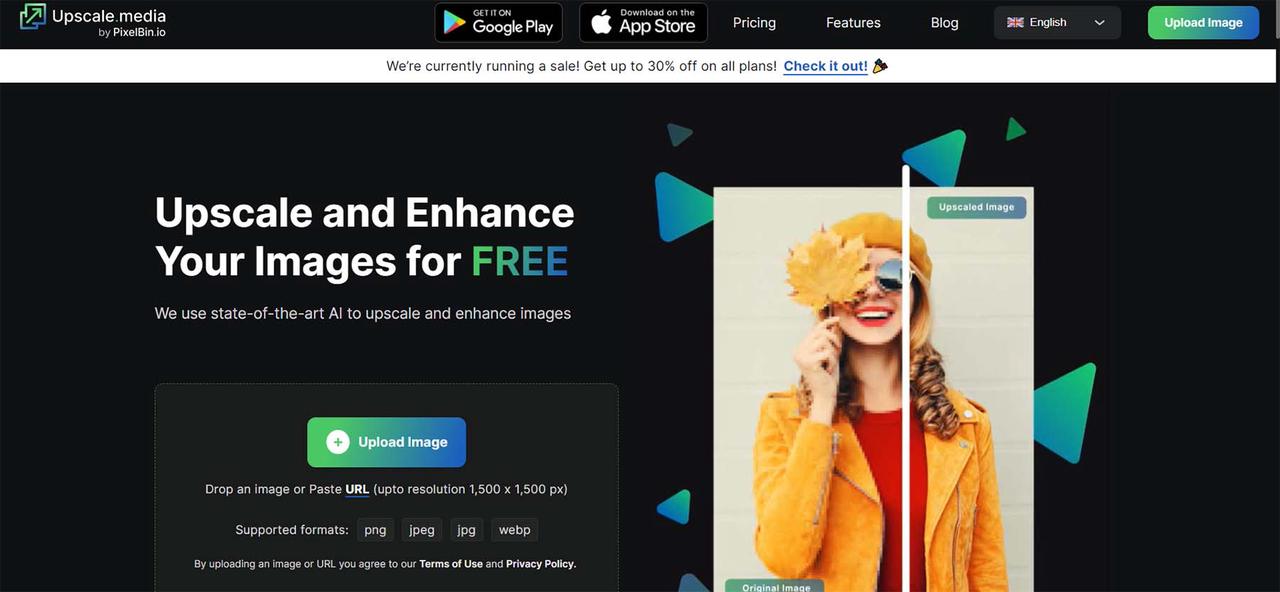The image is a screenshot of a web page titled "Upscale Media," identified by a logo in the upper left corner. The logo consists of a green arrow pointing towards the one o'clock position, encased in a green box with the text "Upscale Media" beside it. Beneath this, in smaller font, it says "pvebin.io". 

Next to the logo on the right, there are buttons for downloading the app from the Google Play Store and the Apple App Store. Adjacent to these buttons are menu tabs labeled "Pricing," "Features," and "Blog," followed by a British flag icon indicating the language setting as English. Further to the right, there is a green button labeled "Upload Image," featuring a subtle blue gradient.

Beneath the menu bar is a white rectangular banner announcing a special sale: "We're currently running a safe sale. Get up to 30% off on all plans. Check it out," accompanied by a blue button with a party hat icon.

The main content of the webpage features a black background with the text "Upscale and enhance your images for free," where "free" is highlighted in a bluish-green color. To the right of this text is an image of a stylishly dressed woman wearing sunglasses and holding a leaf that partially obscures her right eye. To the left is another "Upload Image" button.